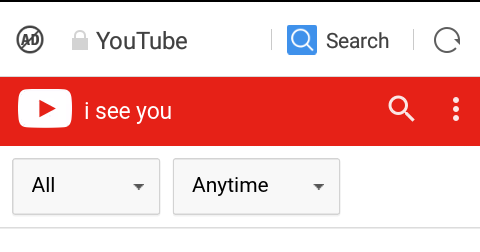A screenshot in front of a white background displays multiple user interface elements. The top section is marked by a horizontal black bar. Below this, "AD" is visible in large text, but it has been struck through, indicating its cancellation or removal. Next to it, the YouTube logo appears prominently accompanied by numerous associated icons.

A distinctive blue square with a white magnifying glass icon signifies a search function or button. Adjacent to this, a refresh button is depicted, likely used to reload the page or content. A vivid red bar stretches horizontally across the screenshot, suggesting a loader or progress indicator.

In the middle section of the image, an outlined white square with a red play triangle inside it denotes a presence of a video element. Further, an "ICU" label in white font is visible, although its context isn't entirely clear.

Additionally, there's another magnifying glass icon, reinforcing the search feature. Three vertical dots, possibly indicating a menu or additional options, are also part of the display. Towards the bottom, two drop-down menus are evident, labeled respectively as “All” with a down arrow and “Any time” with another down arrow, indicating filtering or sorting options.

The screenshot is concluded with a horizontal gray line running along the bottom edge, framing the entire composition. This meticulous synthesis of elements suggests a dynamic interface, possibly of an application or website centralizing multimedia content and optimization tools.